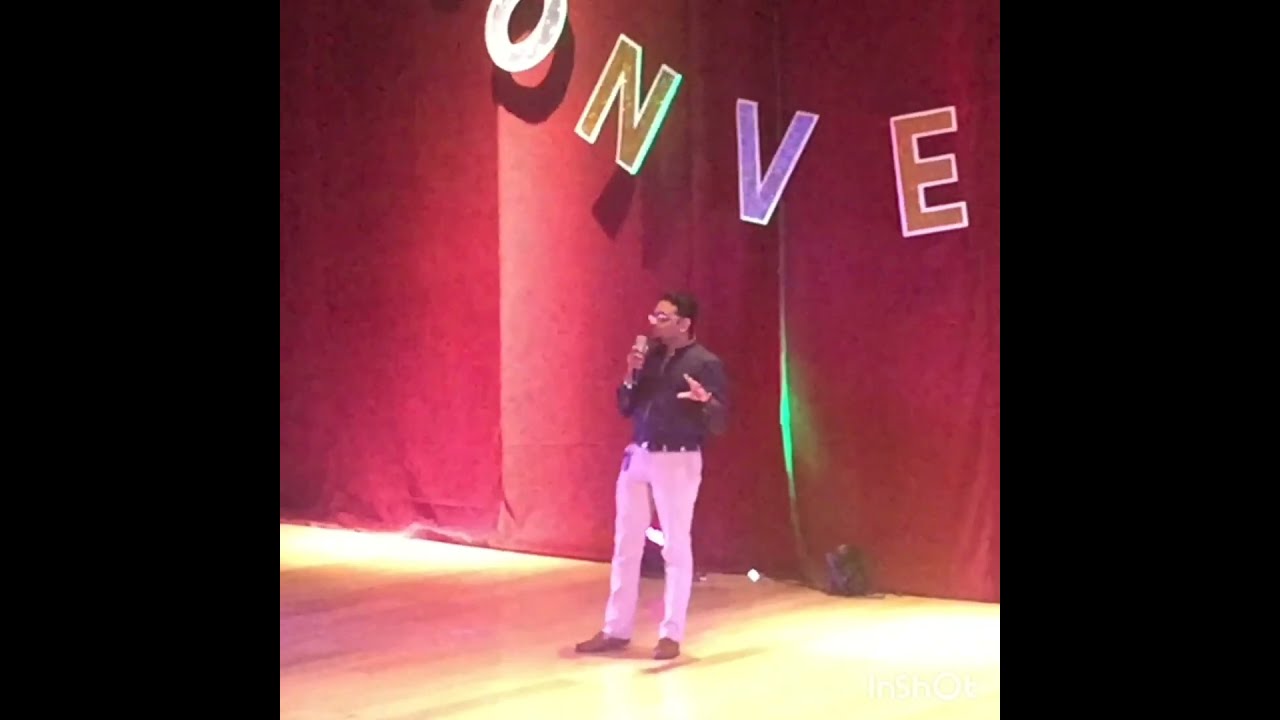In the image, a gentleman is standing on a wooden stage framed by vibrant red curtains. The man, who has black hair and is possibly of Indian descent, appears to be delivering a presentation or speech, as he holds a microphone in his right hand and uses his left hand to make expressive gestures. He is dressed sharply in light-colored pants—variously described as either white or light pink—and brown shoes, identified as either loafers or moccasins. He complements his attire with a black, long-sleeved button-up shirt, which is slightly open at the collar, and a dark belt. Notably, he also sports glasses and appears to have a badge or dark object dangling from his front pocket. A watch may adorn his wrist.

The backdrop of the stage is adorned with the letters O, N, V, and E in white, yellow, purple, and red colors respectively. These letters are illuminated by a small spotlight from below, drawing attention to them against the rich red curtain. A speaker is positioned towards the back of the stage, adding to the setup for his speech. The detailed elements of the man’s attire and the stage setting, including the vivid color palette and the lighting, suggest a formal gathering, potentially a motivational speech or a school event.